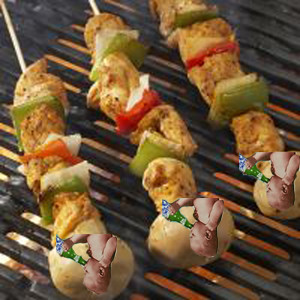The image depicts three shish kebabs grilling over visible flames on black grates. Each skewer is adorned with tan-colored chicken pieces interspersed with vibrant red and green peppers, along with an occasional mushroom. Curiously, at the end of each skewer, there is a peculiar addition: a pale pink rabbit head image, possibly animated or photoshopped, and a small green birthday sparkler with a blue decoration. This unusual detail contrasts with the otherwise traditional barbecue setting, adding a whimsical element to the scene.